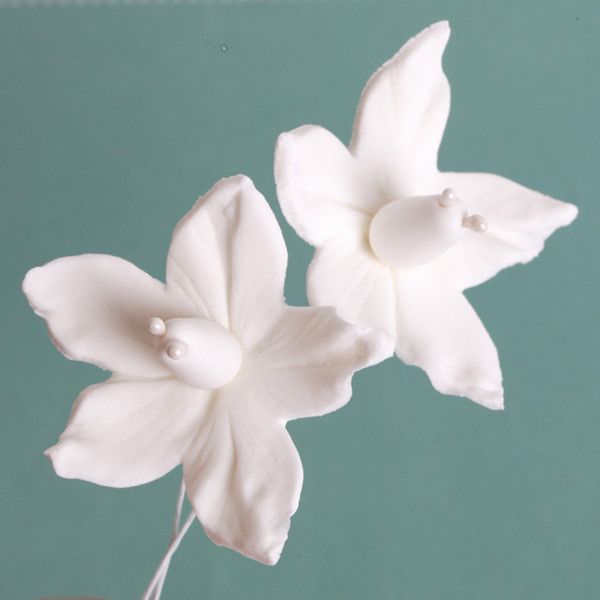The image features two intricately crafted white flowers, seemingly made from edible icing paste. Positioned against a dark turquoise background that gradates from a much darker turquoise in the top left corner to a much brighter shade in the bottom right corner, the scene is delicately illuminated from the right, casting soft shadows. Each flower, perched on thin metal stalks, showcases five substantial petals detailed with pressed vein patterns. The petals reveal their thickness through their pronounced edges. At the center of each flower is a conical structure adorned with two tiny beads protruding from the top, likely affixed to the wire, adding a touch of realism to the edible art.